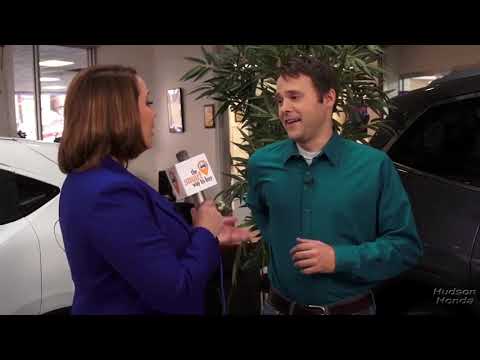In this detailed photograph taken indoors, a woman with shoulder-length brown hair, styled in a bob, is interviewing a man. She is wearing a blue suit jacket and holds a microphone while facing to the right of the image. The man, a white male with short brown hair, is dressed in a green long-sleeve collared shirt and a brown belt. He is standing opposite her and appears to be engaged in conversation, with his mouth open.

The setting suggests a car dealership showroom, indicated by the presence of two cars—a white car behind the woman and a black or gray vehicle behind the man. Further details include a green plant and wall hangings in the background, with a couple of glass windows visible behind the white car, revealing another well-lit room. The bottom right corner of the picture features a watermark reading "Hudson Honda" in small gray font. Additionally, there are two horizontal black strips at the bottom of the image.